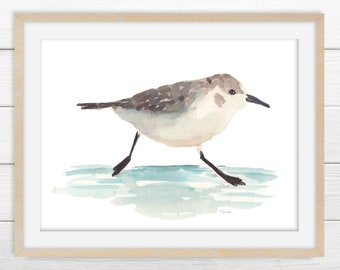The image features a primitive watercolor illustration of a small sandpiper bird running along the shore. The illustration is set against a horizontally slatted white wooden wall. The artwork is framed in natural-colored thin wood and matted with a slightly thicker white border. The bird stands on a patch of ground, depicted in muted tones of cream, light teal, and light gray. The sandpiper has long black legs and a long black beak, with its underside painted in a light cream color. Its wings and head are mottled brown and dark gray, with a distinctive patch of brown on its cheek and dark gray speckles on its top. The bird's eye is black and partially covered by the brown coloring on its head, adding to the primitive charm of the piece. The overall scene captures the delicate and ephemeral nature of the bird and its serene coastal environment.